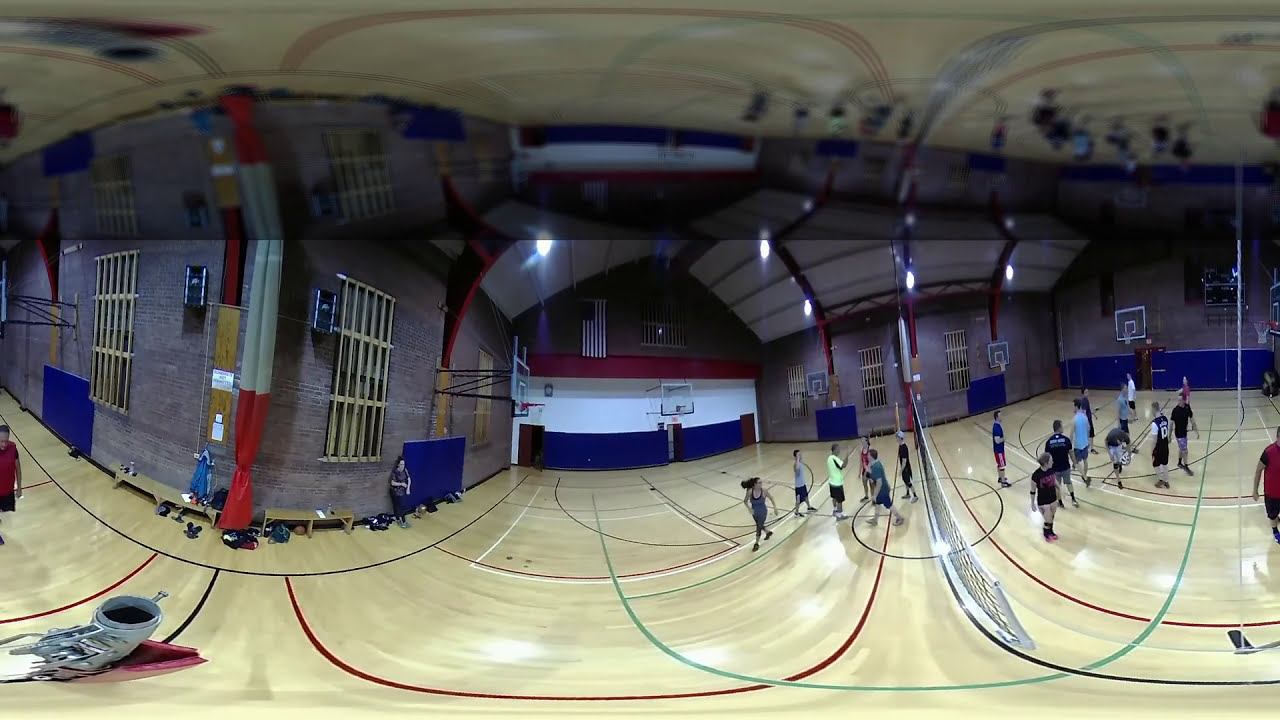This detailed photo, taken inside a gymnasium, showcases a basketball court with a light tan, shiny hardwood floor marked by green, red, and white lines for sports purposes. The scene is slightly warped, suggesting the use of a 360-degree camera, which creates a peculiar curvature and a mirrored effect in the upper half of the image. The court is surrounded by gray brick walls lined with blue padding, clear backboards with white and orange rims, and high windows framed in white for protection.

Several people, dressed in various colors—blue, yellow, red, gray, black—and wearing dark tennis shoes, are engaged in a casual game that appears to be volleyball due to a net spanning the center of the image. Benches are visible against the walls, and the overall setup features scattered positioning of players and objects across the court. The presence of basketball hoops, referees, and possibly younger participants adds to the lively indoor sports atmosphere, although it's unclear whether this was captured during the day or night due to the ambiguous lighting.